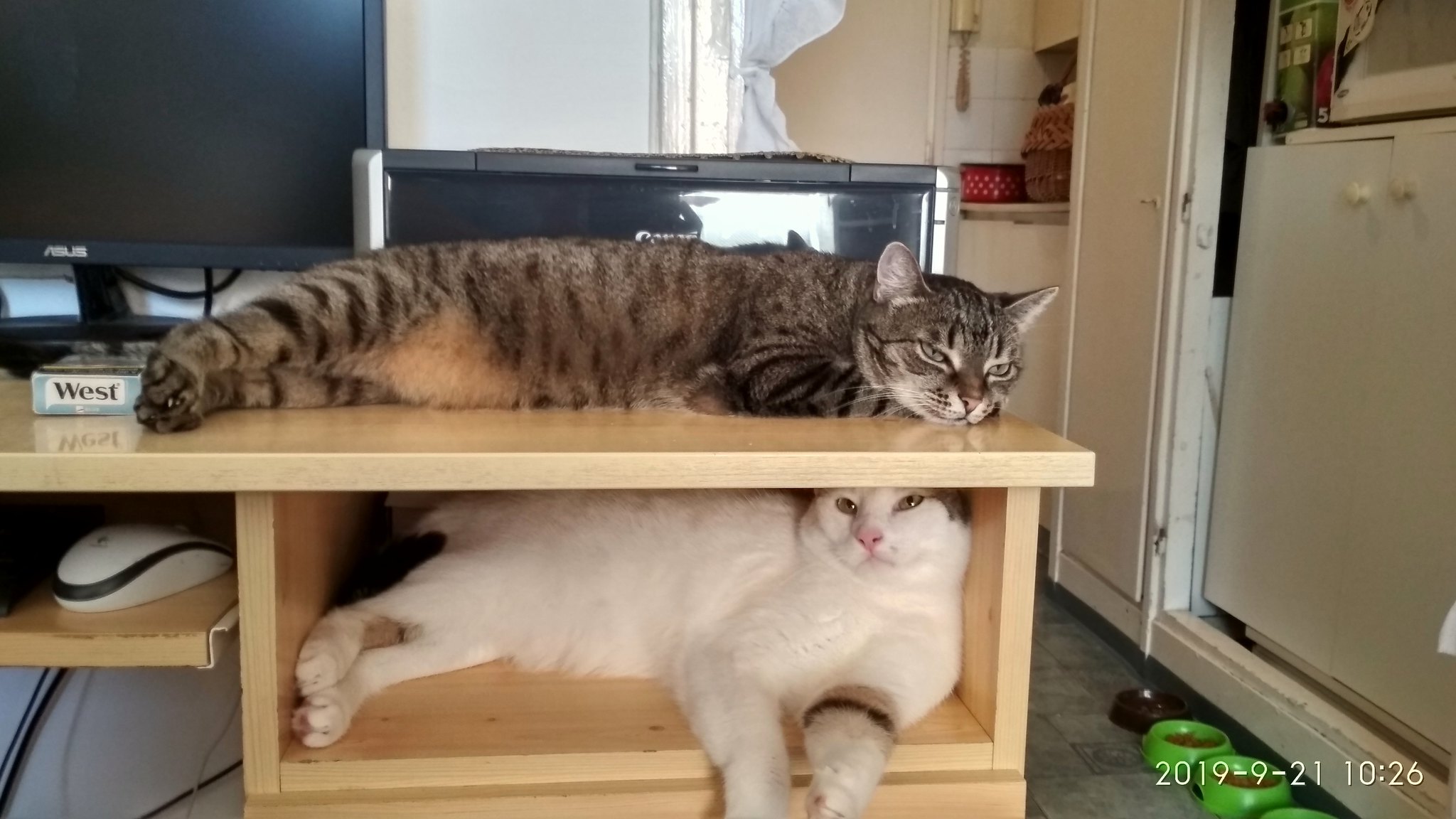The image captures a cozy indoor scene from 2019, depicting a well-organized kitchen setting with a focal point on an entertainment center featuring two adorable cats. The timestamp "2019 921 1026" in white text is visible in the bottom-right corner, indicating the date of the capture. The rectangular photograph, approximately 4 inches tall and 6 inches wide, appears to be taken during the daytime. Central to the image is a light tan wood computer desk with an attached cubby hole. On the top left of the desk sits a black monitor and a printer, both of which are turned off.

Positioned lounging in front of the printer is a relaxed brown tabby cat with distinctive tiger stripes. The cat has its feet extended behind it, front paws tucked beneath its head, and is gazing toward the right. Below the desk, within an empty drawer-like cubby hole, resides a cheerful white cat with a pink nose and slight brown markings on its paws. This cat, with its tail curled behind it and its head squished backward, seems to be looking up knowingly at the tabby cat above.

In the room's background are various elements suggesting daily life, such as cabinets and cupboards. On the tiled floor to the right, there are four cat bowls—three bright green and one black—suggesting meal times are well-organized for the feline companions. The right side of the image shows more storage with white cupboards, adding to the homely and functional ambiance of the space.